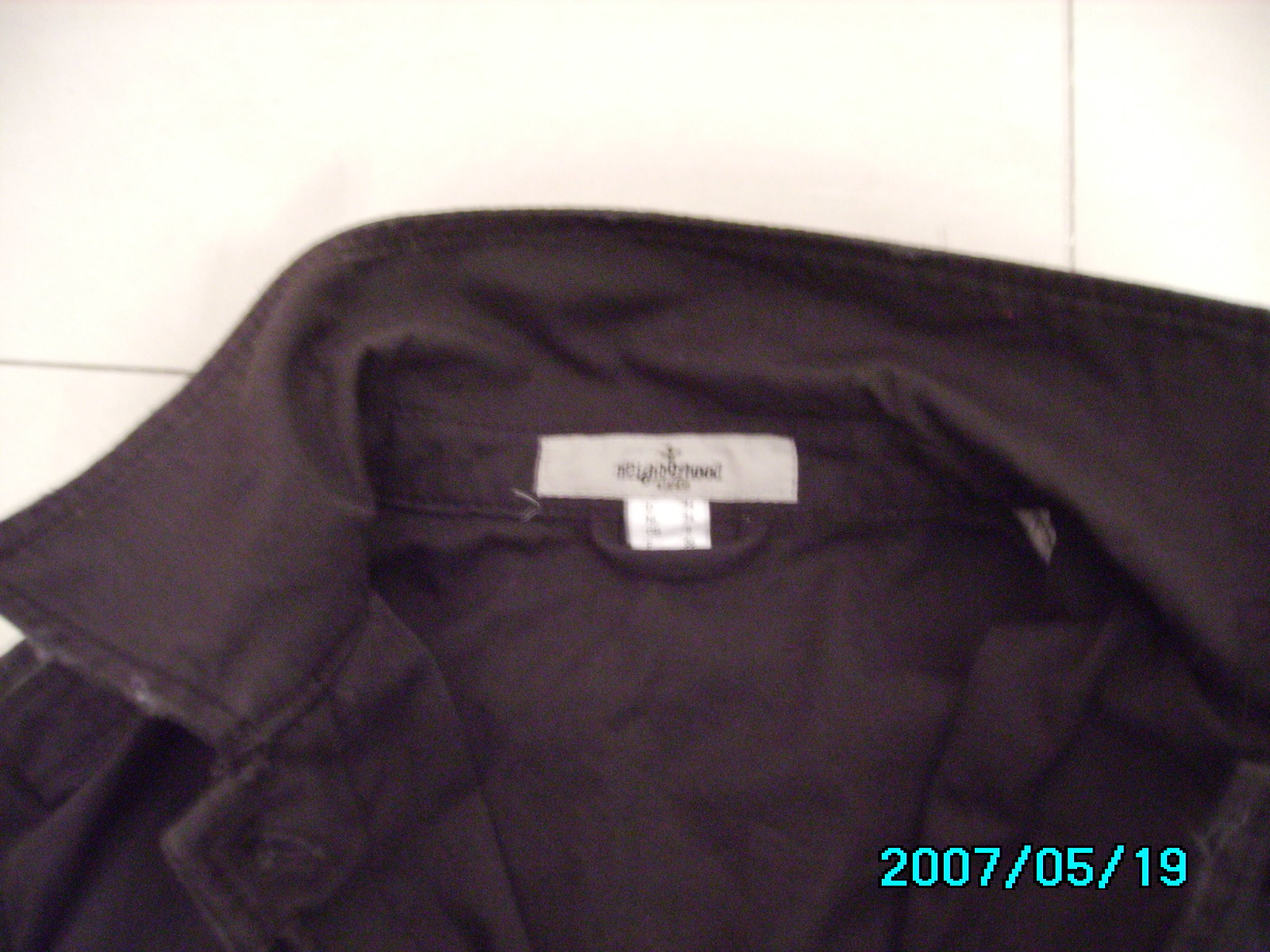The image features an article of clothing, either a jacket or a shirt, predominantly black in color. The garment has a collar that appears slightly pushed up at the back, adding a touch of casual style. Attached to the neckline is a white, rectangular tag, clearly visible despite its small size. From the center of this tag hangs a smaller, square-shaped tag. The larger tag displays the brand name, though the text is too small to discern specific details. On the lower part of the collar's right side, the date "2007/05/19" is printed, adding a unique detail to the garment's design.